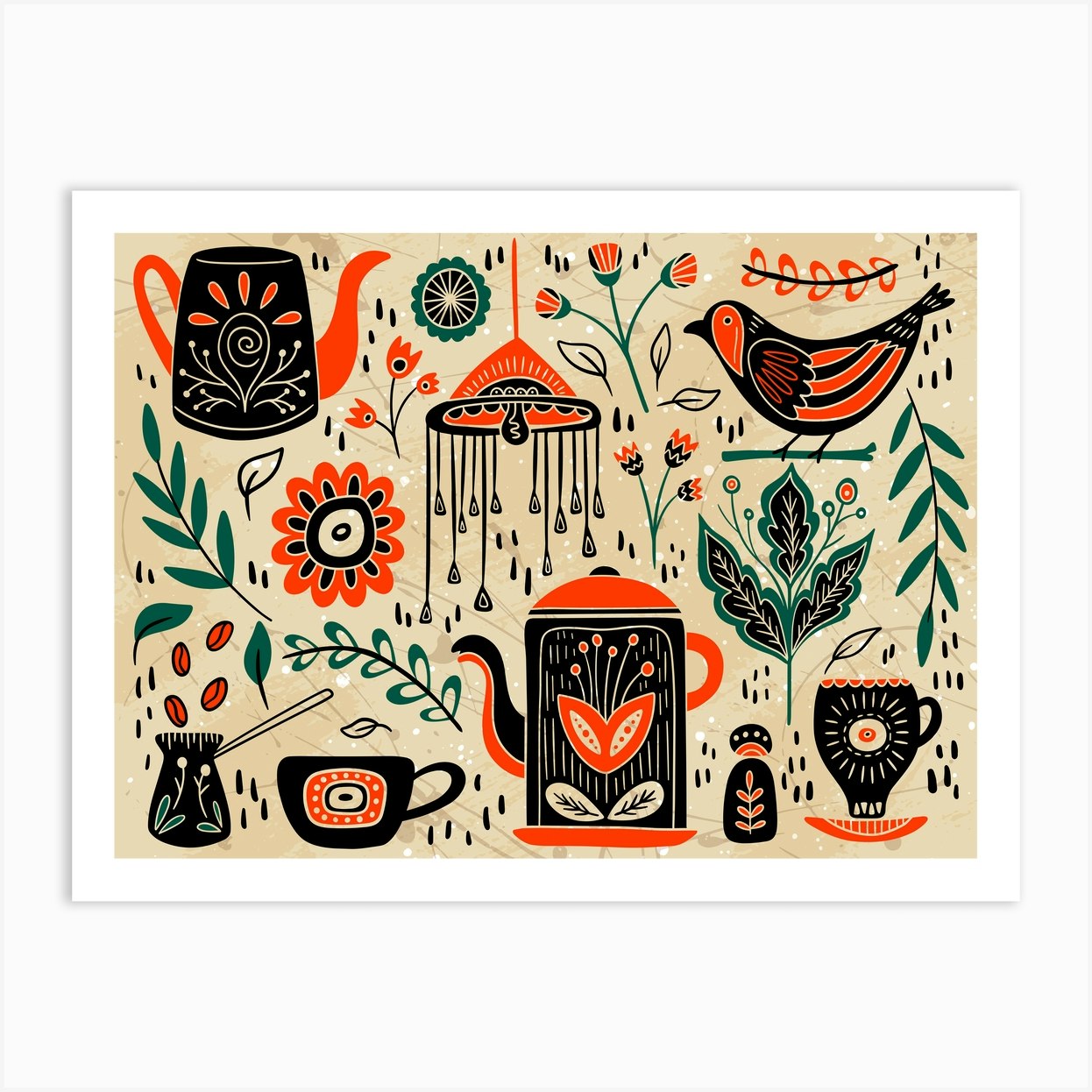The image appears to be a striking piece of artwork designed to resemble a print suitable for framing. It features a light tan background with an intricate pattern of diverse elements that exude a folksy, abstract aesthetic. The perimeter of the image is bordered in white, enhancing its overall sophisticated appeal. Centrally, there is an ornate, chandelier-like structure with decorative hanging elements, surrounded by an array of items. Scattered throughout the composition are various teapots, teacups, a pitcher, and a small vase. The predominant colors are black, orange, green, and burgundy. A coffee mug sits in the bottom right corner, depicted in black, conveniently positioned next to an orange peel and a large black-and-orange pitcher. The upper right corner houses a bird sporting red and burgundy hues. The entire scene is interwoven with beautifully painted leaves, flowers, twigs, and branches, adding to the lively yet harmonious arrangement of the artwork.